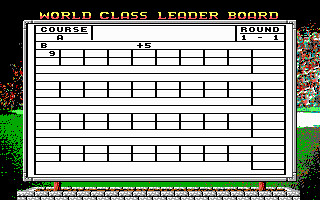The image depicts a vintage video game leaderboard screen, possibly from a classic Nintendo or similar console game. The display features a rectangular white board set within a stone-like base, complete with red posts on either side. At the top, on a black background, yellow and red letters spell out "World Class Leader Board," indicating the title of the leaderboard. Below this title, the board is divided into a grid with multiple rectangular spaces intended for scores.

The first row is labeled "Course A" and "Round 1 of 1," setting the context for the competition. Within the grid, the first column in each section has the letters "B" and "9" prominently displayed, alongside a "plus 5". The grid is structured to accommodate ten scores per section, with lines that divide it into four distinct groups of ten blanks each. The background features a green grassy area suggesting an outdoor setting for a sporting event. The detailed layout and labeling of the board makes it clear that it is designed to track and display multiple scores for various rounds and courses.